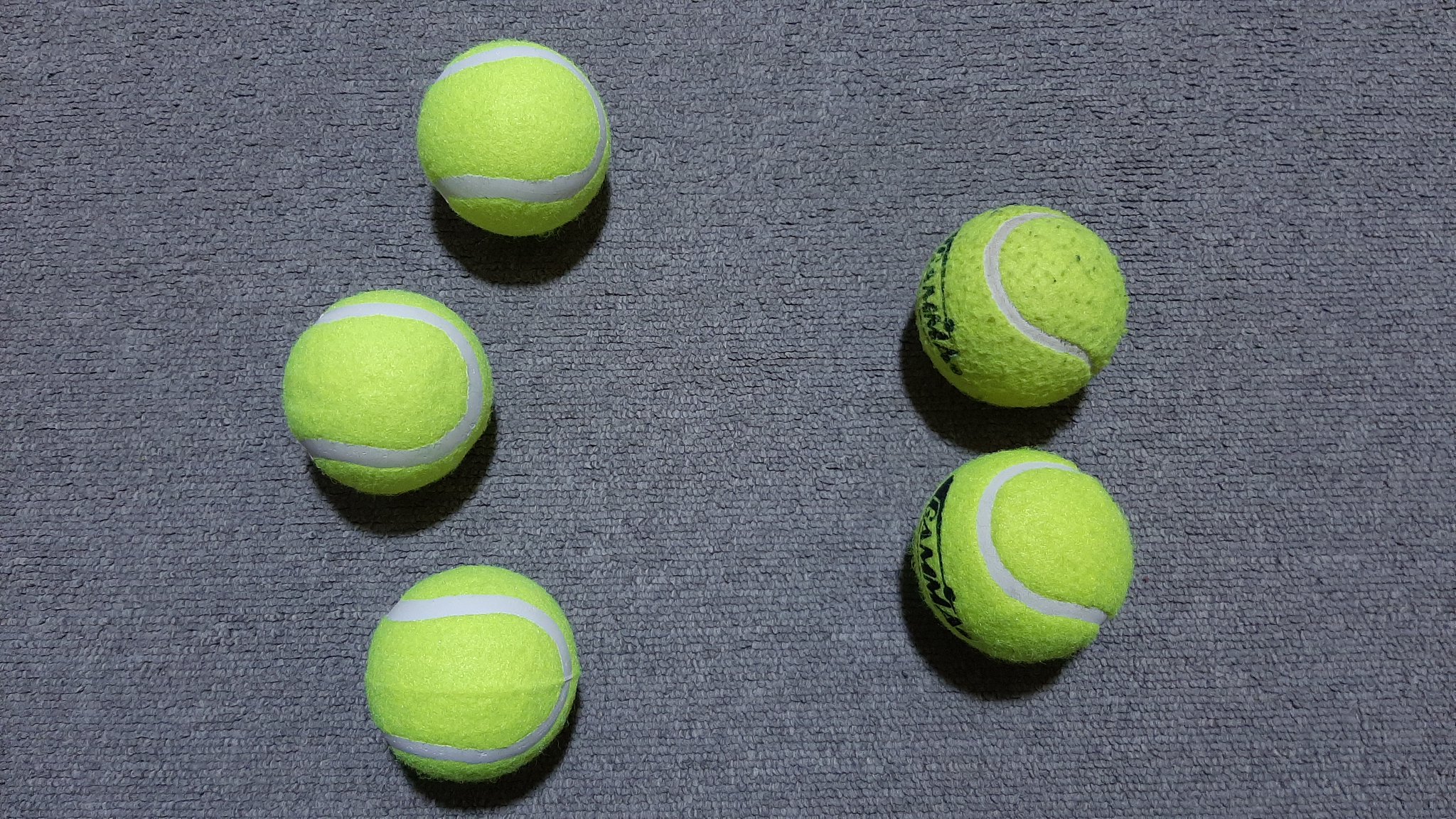This landscape photograph captures an overhead view of five light green tennis balls, each adorned with a distinctive white curving seam, resting on a textured dark gray carpet that resembles an office floor. The short fibers of the carpet appear pressed down in spots, contributing to a smooth, flat appearance. The tennis balls are positioned in two distinct groups: three on the left and two on the right. The trio on the left is arranged in a slight V-shape or small triangle, with one tennis ball slightly offset. The pair on the right is aligned vertically, one directly above the other, about an inch apart. Both of these right-side tennis balls feature a black logo, though the text is obscured from this angle. Shadows cast by the tennis balls form crescent shapes on the carpet, and one ball, in particular, exhibits signs of wear, including smudging and black streaks. The overall hue of the tennis balls—an ambiguous light lime green or fluorescent yellow—may shift slightly due to the lighting in the photograph.